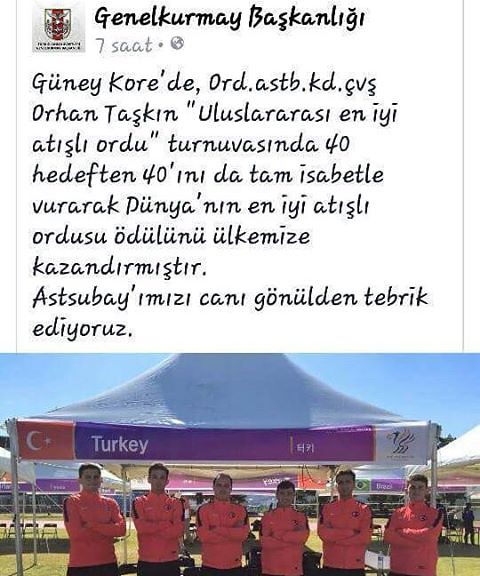The image depicts a close-up of a social media post showcasing a sports team from Turkey. The post begins with text in Turkish, which is not legible, and features a rectangular image of a gazebo with a white top. The image prominently displays a purple banner with the word "Turkey" in white letters, accompanied by the Turkish flag—a red background with a white crescent moon and star. To the right of the flag, there is an additional white square containing gold and dark blue squiggles, possibly a logo. The team consists of six men, all wearing pink windbreakers and black pants, standing side by side under the gazebo on a sunny day. They are posed with their arms crossed, smiling at the camera. Behind them, there are more gazebos of the same design, folded chairs, and other individuals, all set against a backdrop of green grass and a clear blue sky, suggesting a festival or gathering atmosphere.